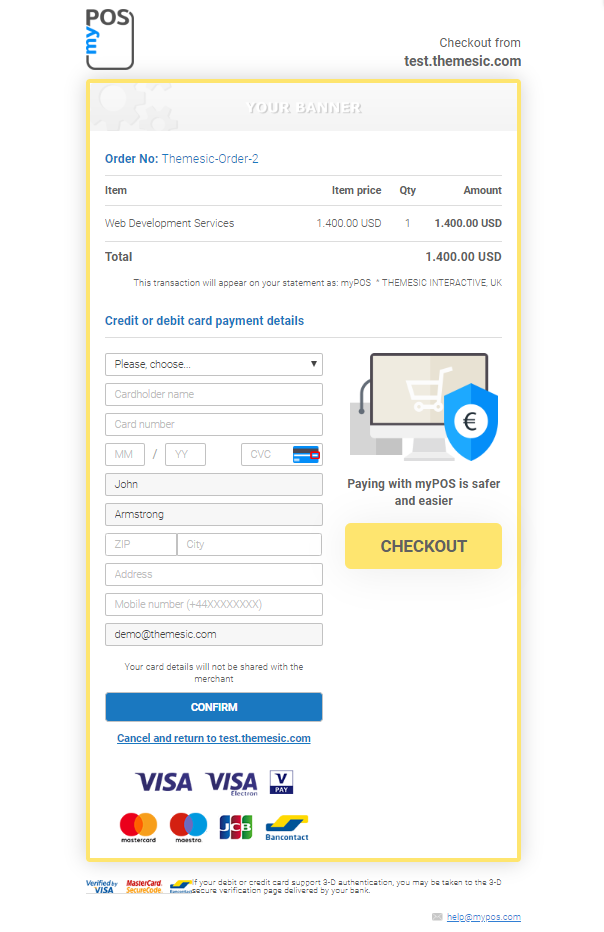This image depicts an interface mockup for an online payment checkout system. At the topmost inch, the image is white. Below this, there is a yellow border that surrounds the bottom section, extending an inch into the top of the frame. Inside the yellow border, the background is light gray until it transitions to white.

In the top-left corner of the white section, the text "MY" is vertically aligned along the left edge, and "POS" is horizontally aligned across the top. A line runs down the right side and continues beneath the bottom edge of the white area. In small black lettering along the bottom right, it says, "check out for form"; slightly larger, it reads "test themastic.com."

Within the yellow border on a blue background, the text "your banner" is displayed above an order number. Below this section, there are columns for "Themes" and "Orders." Underneath these headings, the left side lists an "Item" and its corresponding name, while the right side includes the "Amount" and the cost. To the left of the amount is "QTY," under which the quantity of items is indicated, followed by "Item Number."

At the bottom left is a section labeled "Total." Next, in blue text, it states "Credit or Debit Card Payment Details." This part includes fields for various credit card details. To the right, there is an image of a computer monitor displaying a shopping cart icon, a blue shield with a white circle and an 'E' symbol split by two lines. Below this, in black text, it says, "Paying with my POS is safer and easier."

At the bottom of the credit card information section, there is a yellow tab with the word "Check out" in black. Beneath this tab, there is a blue button that says "Confirm" in white text. At the very bottom, there is a list of all the different credit cards that are accepted.